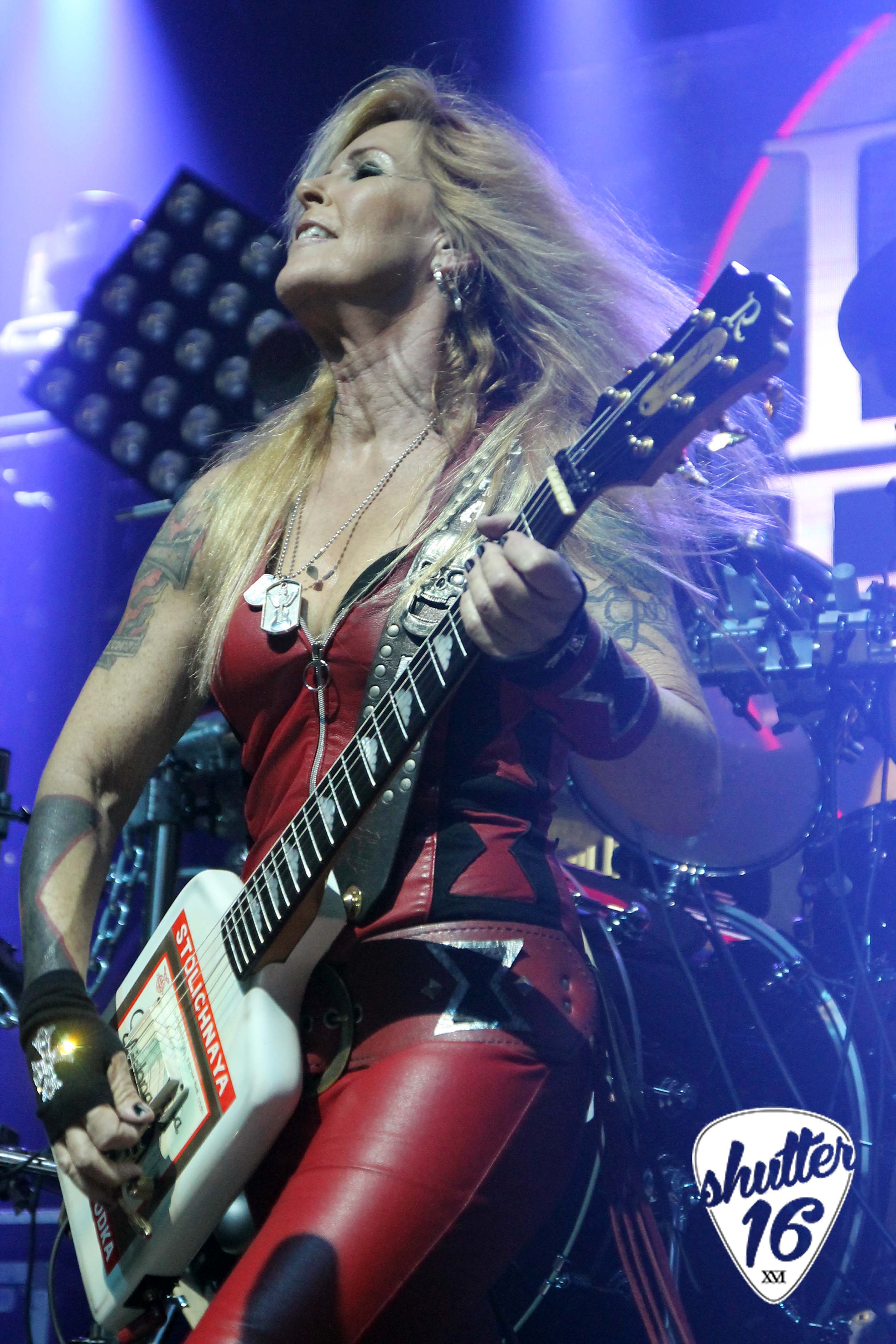This dynamic photograph captures a powerful female rock star, possibly Lita Ford, mid-performance on stage. She sports an eye-catching red leather ensemble comprising tight red leather pants cinched with a prominent red belt and a matching red tank top-style top with a central zipper. Her long, flowing blonde hair cascades back, enhancing the sense of motion in the image. Tattoos adorn both her arms, adding to her rock 'n' roll persona. Around her neck, she wears a chain with dog tags, while her right hand is clad in a black fingerless glove decorated with a silver cross, potentially encrusted with gems. In both hands, she firmly holds a unique square-shaped guitar, predominantly white with black accents and emblazoned with the word "Stolichnaya," resembling a vodka bottle in shape. The stage lighting casts a dramatic blue hue from the upper left, while a drum set is partially visible behind her. In the bottom right corner, a white guitar pick-shaped logo features blue text reading "Shutter 16." The photo exudes energy and showcase a seasoned rock star in her element.